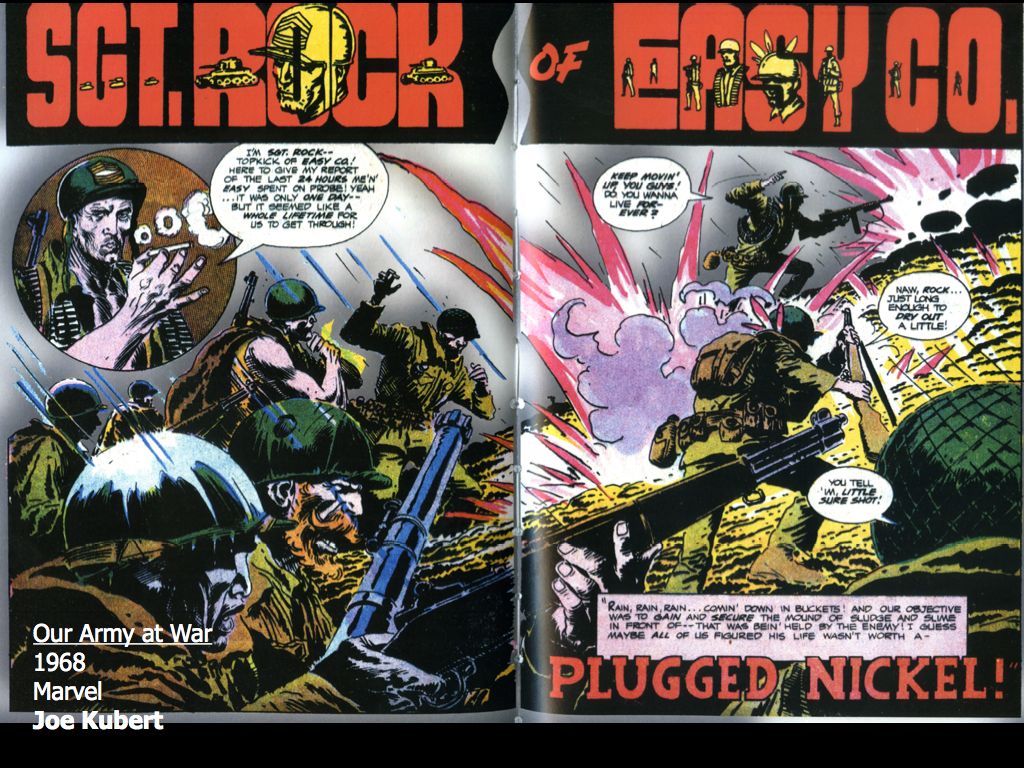The image is a two-page spread from a vintage comic book titled "Sgt. Rock of Easy Company." It appears as a continuous war scene despite the visible central border and staples. At the top, large red letters spell out "Sgt. Rock of Easy Co" against a stark black background. The pages are filled with dynamic illustrations depicting soldiers in the throes of battle, complete with rifles, helmets, and intense expressions. Explosions and chaotic scenes dominate the artwork, with numerous soldiers advancing and engaging the enemy.

In the lower left corner, a soldier is shown firing his rifle, the barrel extending into the opposite page, which further emphasizes the cohesive flow of the scene. Speech bubbles scattered throughout feature dialogue typical of war comics, including motivational and gritty exchanges among the soldiers. One inset in the upper left corner shows a commander, presumed to be Sgt. Rock, smoking and delivering a speech. The text reads, "I'm Sgt. Rock, Topkick of Easy Co, here to give my report of the last 24 hours. Yes, it was only one day but it seemed like a whole lifetime for us to get through." Another soldier's bubble reads, "Keep moving up you guys, do you want to live forever?" with a response, "Nah Rock, just long enough to dry out a little."

At the bottom of the pages, small text notes the comic is from "Our Army at War," dated 1968, Marvel, with the author cited as Joe Kubert. A description adds, "Rain, rain, rain coming down in buckets and our objective was to gain and secure the mound of sludge and slime in front of us being held by the enemy. I guess maybe all of us figured his life wasn't worth a plugged nickel."

Overall, the detailed artwork and evocative text paint a vivid and intense picture of a day in the life of Sgt. Rock and his company.